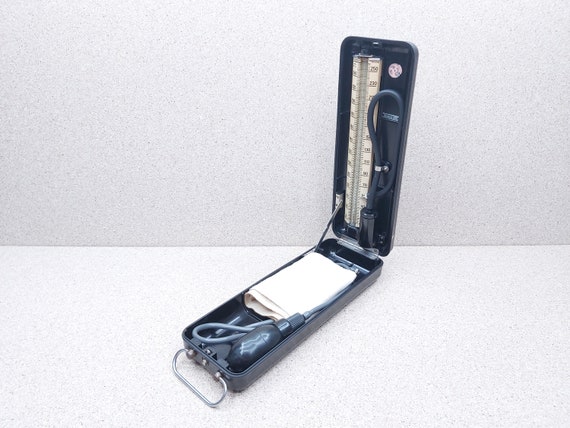This close-up photograph showcases an antique blood pressure machine from the 1950s or 60s. The device is enclosed in a dark blue, rectangular case with a gray steel handle on the left side. The case is open, allowing a clear view of the contents inside. On the left side of the case, there is the blood pressure cuff and the air pump, commonly known as the squeezer, both in dark blue, and a white napkin positioned nearby. The pump connects to a central blast cylinder, which is flanked by numerical markings for blood pressure readings on either side. On the right side, the mechanism attaches to a vertical, thermometer-like gauge with a red line indicating the blood pressure readings. This setup rests on a gray and white speckled countertop with a similarly colored background, highlighting the vintage and utilitarian design of the medical equipment.